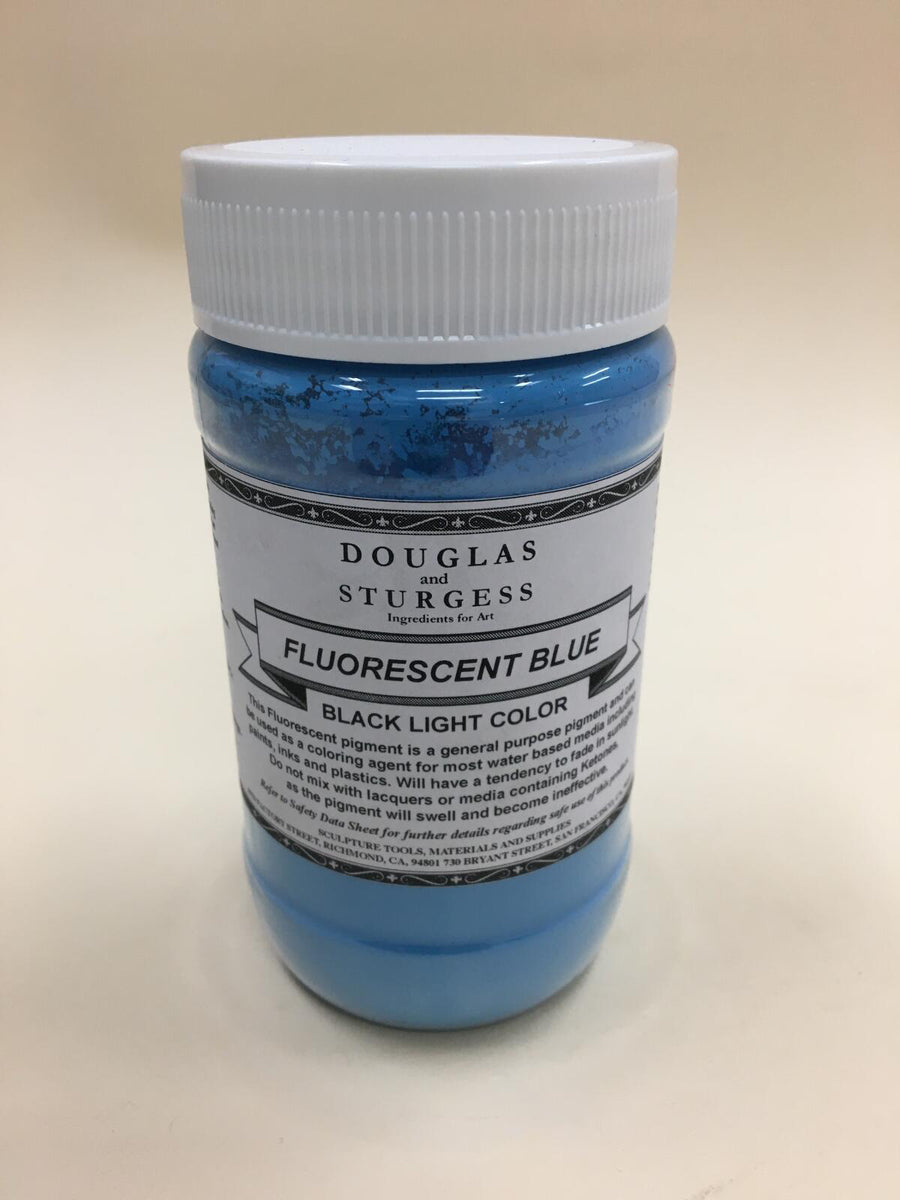This is a close-up photograph of a small clear plastic jar, approximately 7 to 8 inches tall, containing a vibrant blue pigment. The jar is capped with a tightly twisted white lid that has ridges around its edge. The blue pigment inside appears solid at the bottom, with some darker areas near the top, suggesting the jar is not completely full. The jar is set against a beige, off-white background.

Affixed to the jar is a white label with a black border at the top and bottom. The label displays the text "Douglas and Sturgis, Ingredients for Art" in black. Below this, a ribbon-like design bears the words "fluorescent blue," followed by "black light color." The lower section of the label contains further information, although the fine print is somewhat blurred and wraps around the jar, making it difficult to read entirely. This text indicates that the product is a general-purpose pigment suitable for use in lacquers or other media, and is specifically designed to glow under black light, producing a fluorescent blue color.